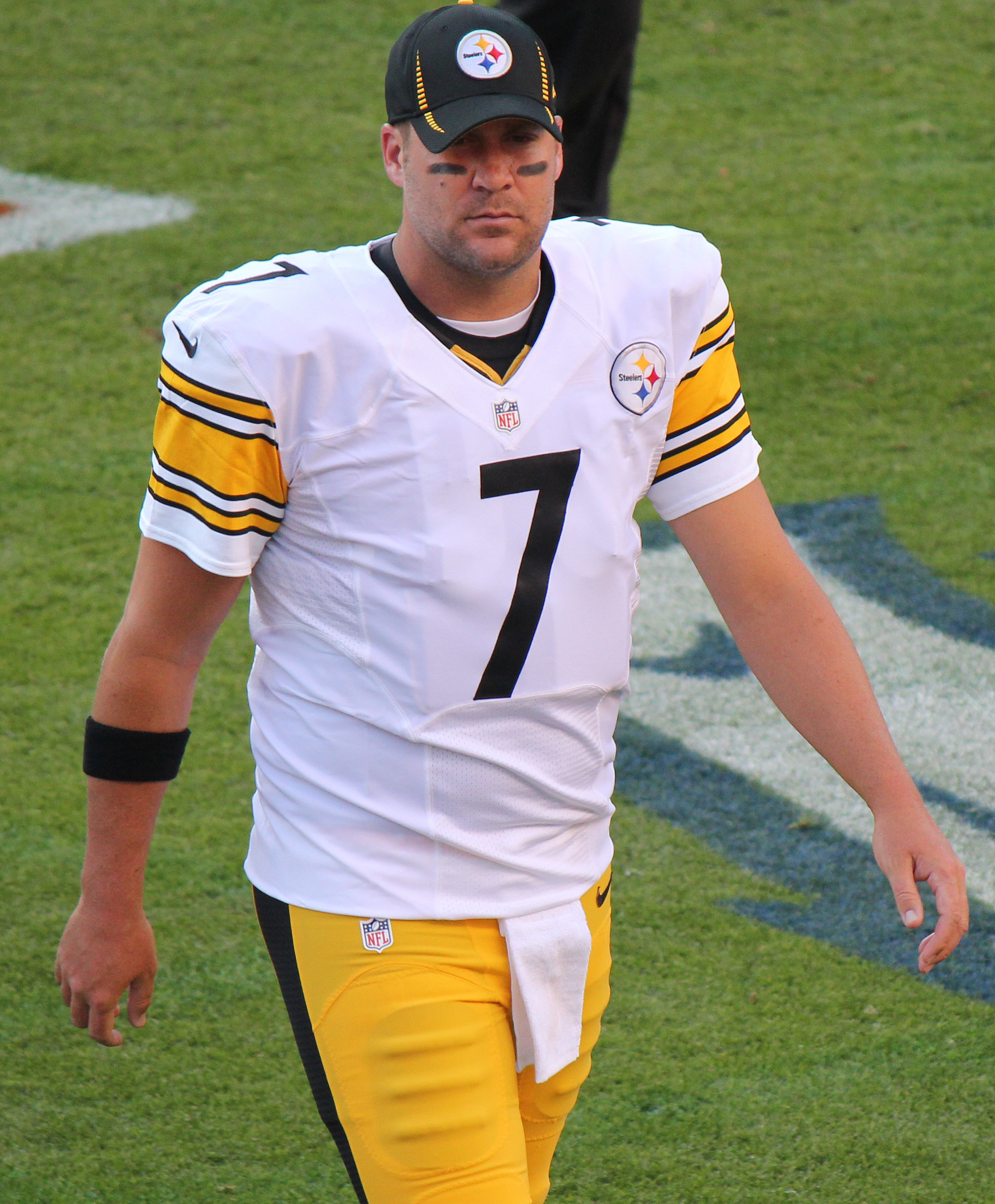This close-up photo captures future Hall of Fame quarterback Ben Roethlisberger of the Pittsburgh Steelers walking towards the camera on a football field. Roethlisberger is wearing the Steelers' distinctive white jersey, which features his black number 7 prominently on the chest, flanked by the Steelers logo near his left shoulder and the NFL logo on the v-neck. His short sleeves are detailed with yellow bands and black number 7s, accompanied by a Nike swoosh on his right shoulder. Completing his look, he's also adorned in yellow pants with a black stripe running up the leg, accessorized with a white towel displaying the NFL logo and a Nike swoosh. Roethlisberger sports black face paint under his eyes and a black Steelers ball cap with the team logo in the center. In the background, a small portion of another player's leg is visible, clad in black pants, hinting at the presence of teammates.